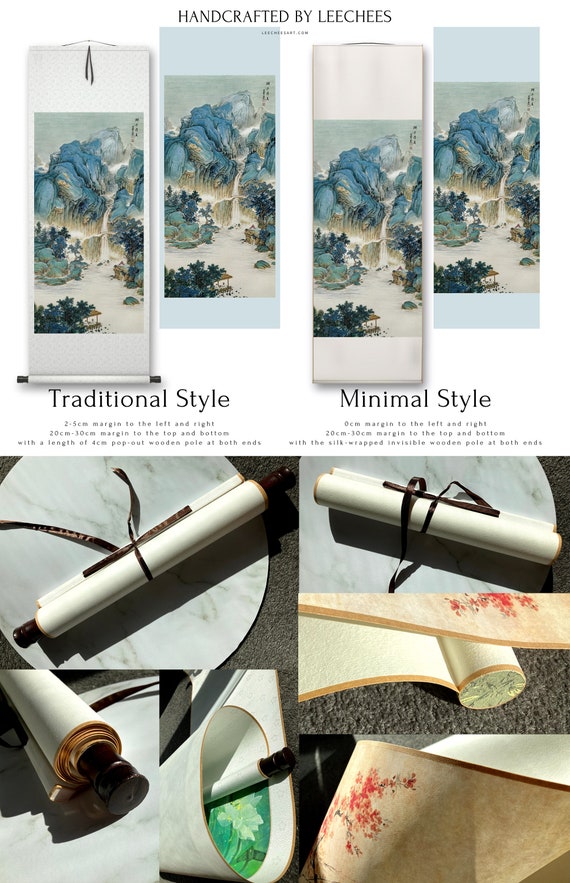This promotional image showcases Japanese products, divided into distinct sections. At the top, the brand "Handcrafted by Leach Ease" is prominently displayed, indicating the maker or company. This section features two styles of scrolls: one labeled "Traditional Style" and the other "Minimal Style." Both have a white and light blue background with rocky landscape imagery depicting mountains, rivers, waterfalls, and trees. However, no additional text describes the actual products. 

In the lower half, multiple photographs are shown. These images illustrate the scrolls when fully unrolled, highlighting their texture and intricate designs. Some photos depict the scrolls rolled up, much like traditional Chinese or Japanese picture scrolls, designed for easy storage or wall display in a domestic setting. The bottom section also includes items like a paint pot with green paint and what appears to be a piece of wrapping paper used for cleaning the paintbrush.